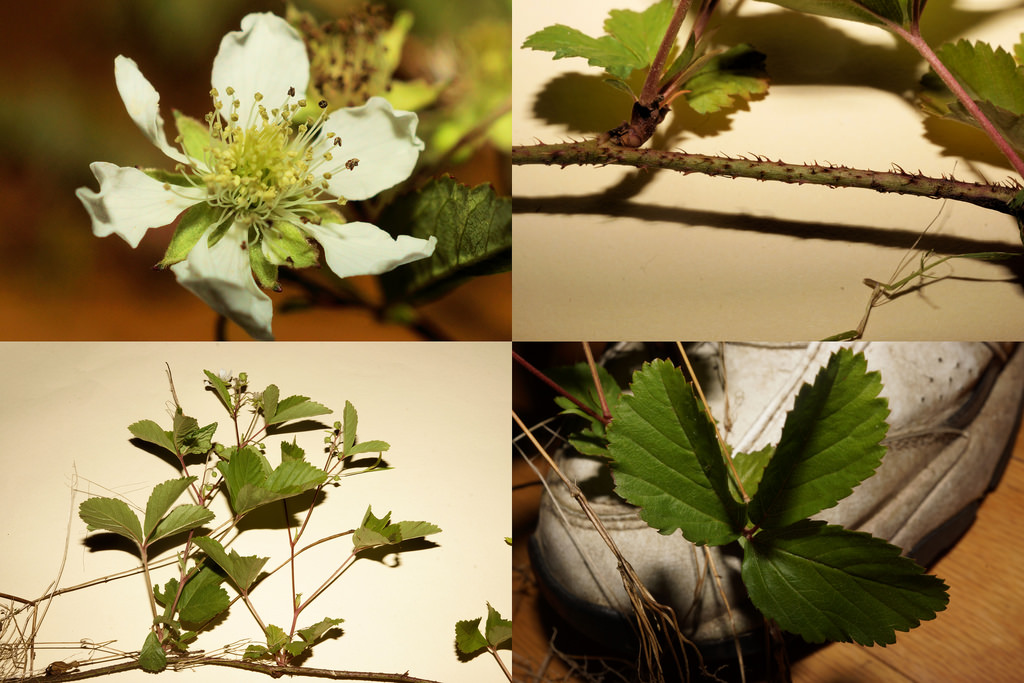The image comprises a collage of four landscape-oriented photographs, each depicting different parts of a berry bush. The top left photo captures a close-up of a white blossom with six petals radiating outward and a center filled with delicate, light green stamens. Behind the flower, a slightly curled green leaf is visible against a blurred background. The top right photo displays a green stem punctuated with small red thorns, and two blossoms emerge from this thorny stem. The bottom left photo showcases the main branch of the plant with multiple green leaves extending from it, while the bottom right photo offers a detailed close-up of the green foliage, highlighting the leaf structure. All elements are presented with photographic realism, focusing on the plant's intricate details.